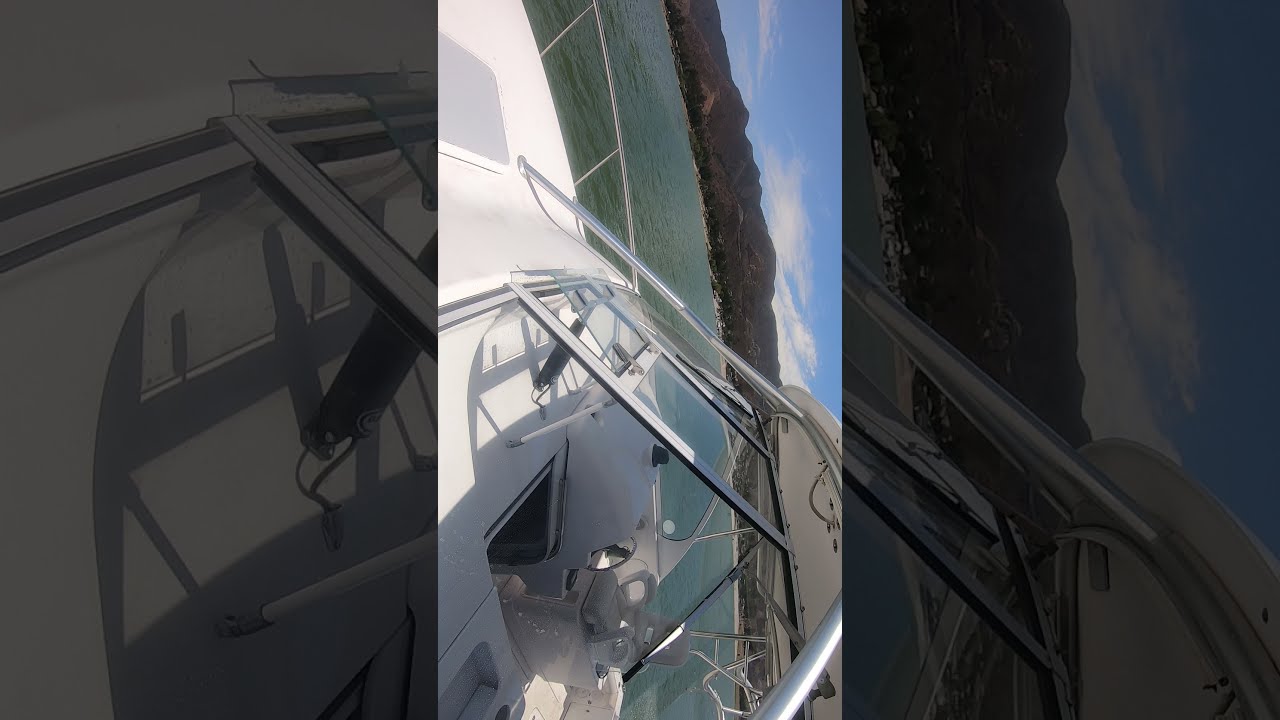This is an image of a small, white motorboat turned sideways, requiring a tilt of the head for proper viewing. The boat, featuring a canopy and silver railing, floats on calm, teal-green water with minimal ripples. It has a small glass windshield and seating for one person, though the cockpit remains empty, suggesting it might be parked. The photograph, transposed on top of itself, creates a mirrored effect, vertically slicing the image in the center. This vibrant central slice contrasts with the darker, faded edges. The background showcases a serene landscape, including a sandy beach, verdant green trees or shrubs, and distant grayish mountains with hints of greenery. Above, the sky is a bright blue adorned with a few wispy white clouds, indicating a clear, beautiful day.